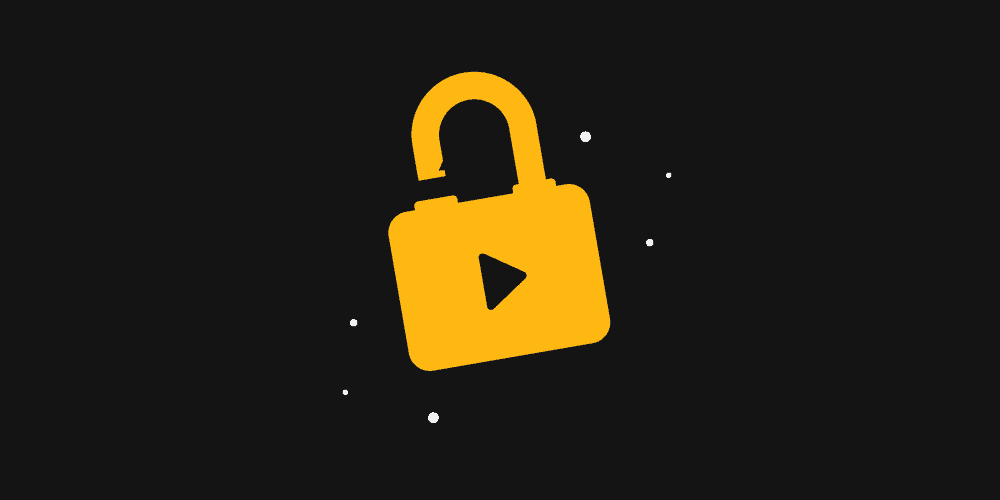The image is a color illustration designed in a simple, minimalist style with a flat, 2D appearance and three colors. It has a landscape orientation, making it a wide rectangle with the top and bottom sides twice as long as the left and right sides. The background is solid black, while the central figure—an outline of an unlocked padlock—is depicted in a yellowish-orange hue. The padlock is partially open, creating a small gap on its left side. The front of the padlock features a black cutout in the shape of a right-facing triangle, resembling a play button. Additionally, there are three white dots on the bottom left and three more on the top right of the padlock, hinting at movement or energy. No text accompanies the image. This piece likely conveys a theme of security or access, using its stark color contrast and clean lines to draw attention to the central unlocked padlock.